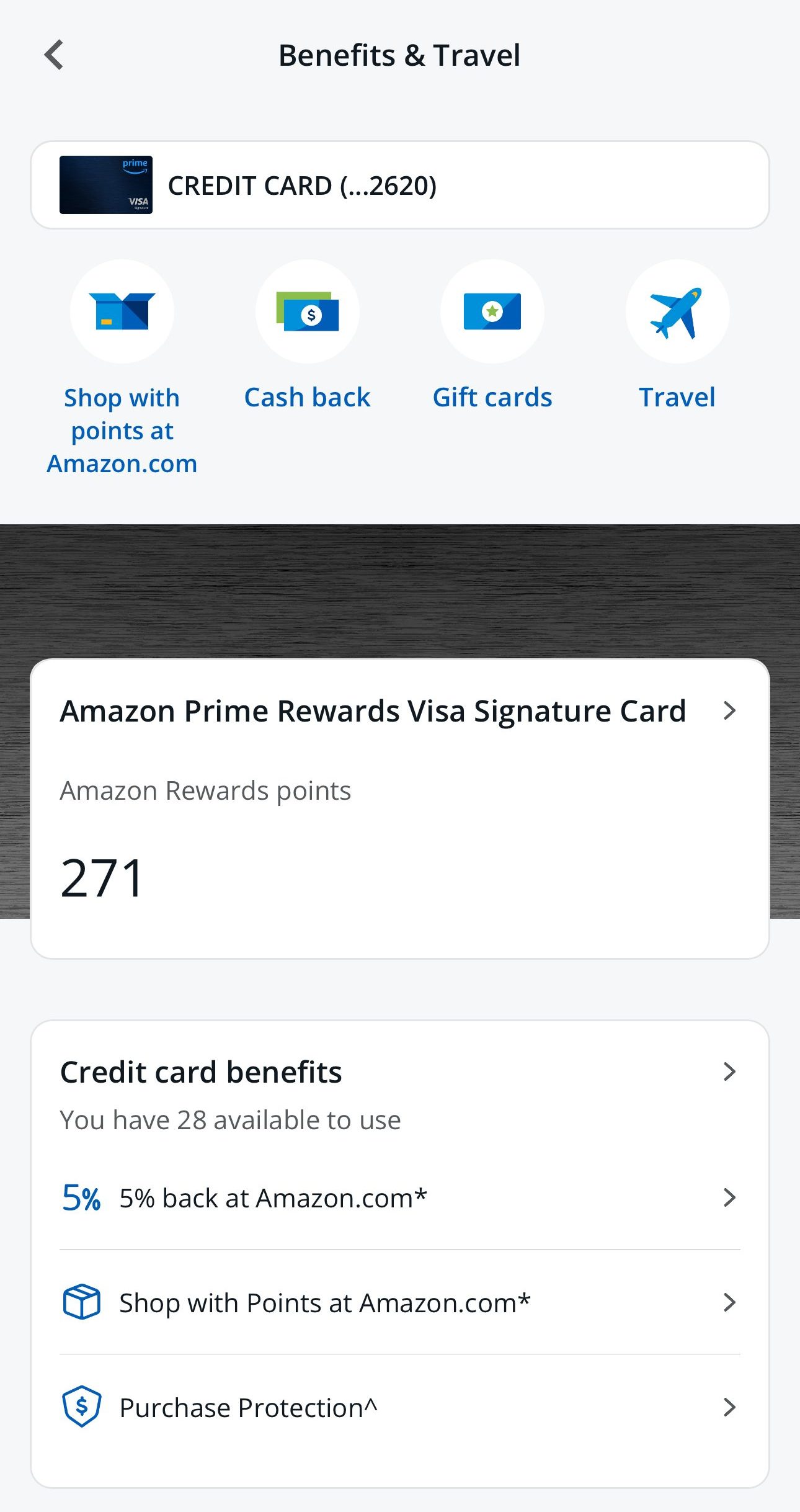The image depicts a credit card rewards page focused on benefits and travel. At the top of the page, the header displays "Benefits and Travel" with a back arrow. Below the header, the credit card information is partially shown with the last four digits 2620.

The page is populated with various icons and buttons. The first icon represents the option to "Shop with Points at Amazon.com" and features a blue open box. Adjacent to this, the "Cash Back" option is illustrated with a green and blue dollar bill icon that has a dollar sign in its center. The third option, "Gift Cards," is symbolized by a blue envelope adorned with a green star. Finally, the "Travel" option is depicted by a blue airplane icon.

Further down, the page provides specific details about the user's card: the "Amazon Prime Rewards Visa Signature Card" with "Amazon Rewards Points: 271." There is also text indicating "Credit Card Benefits" available to the user, noting that there are 28 benefits with an arrow prompting further exploration. Each benefit is listed with small black arrows behind them. The listed benefits include "5% Back at Amazon.com," "Shop with Points at Amazon.com," and "Purchase Protection."

The overall layout of the page has a primarily white background, but the central area, which highlights the credit card details, is rendered in a darker black color that resembles the design of a credit card.